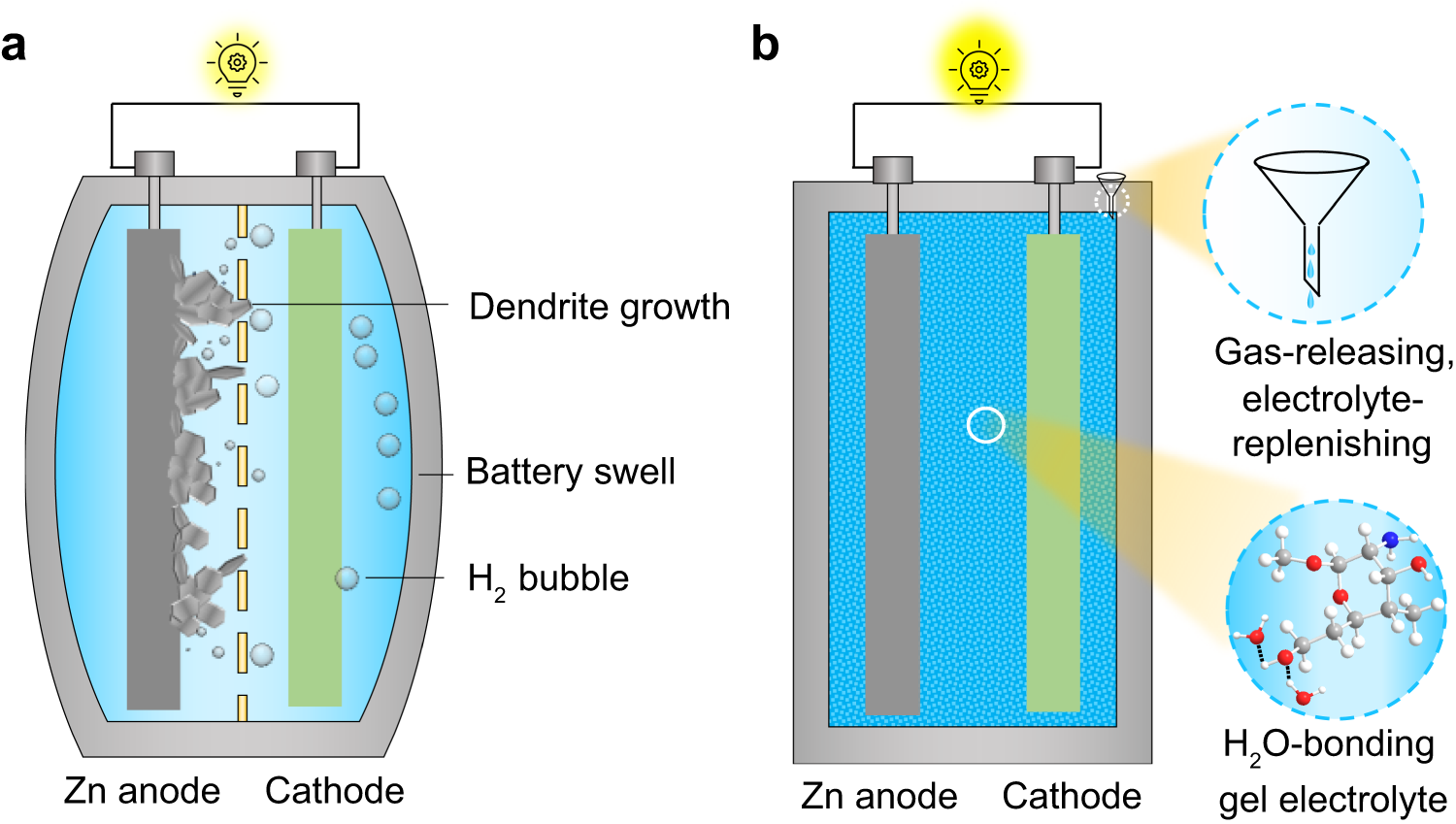The scientific diagram on a white background features two illustrations labeled A and B, showing cross-sectional views of batteries. Both images have a yellow light bulb at the top, with battery A emitting a dull yellow light and battery B displaying a vibrant, strong yellow light. Illustration A is of a barrel-shaped battery, while B depicts a square-shaped battery.

In battery A, the gray outline shows a bulging form with two cylindrical components running vertically from top to bottom— a thick gray line on the left and a thick green line on the right. Inside battery A, callouts highlight "dendrite growth" near the top, "battery swell" on the outer side, and "H2 bubble" near the green line. The lower part identifies the components as "Zn anode" on the left and "cathode" on the right.

Battery B shares similar internal elements, including a gray and green line on the left and right, respectively. This battery also includes a white circle in a blue background at the center, labeled "H2O bonding, gel electrolyte." Additionally, it features a funnel-shaped object with labels "gas-releasing" and "electrode-replenishing," showcasing its sustainability attributes. Battery B's lower part is also labeled "Zn anode" on the left and "cathode" on the right. The diagram emphasizes the contrast between battery A's problematic features and battery B's sustainable, healthier design.